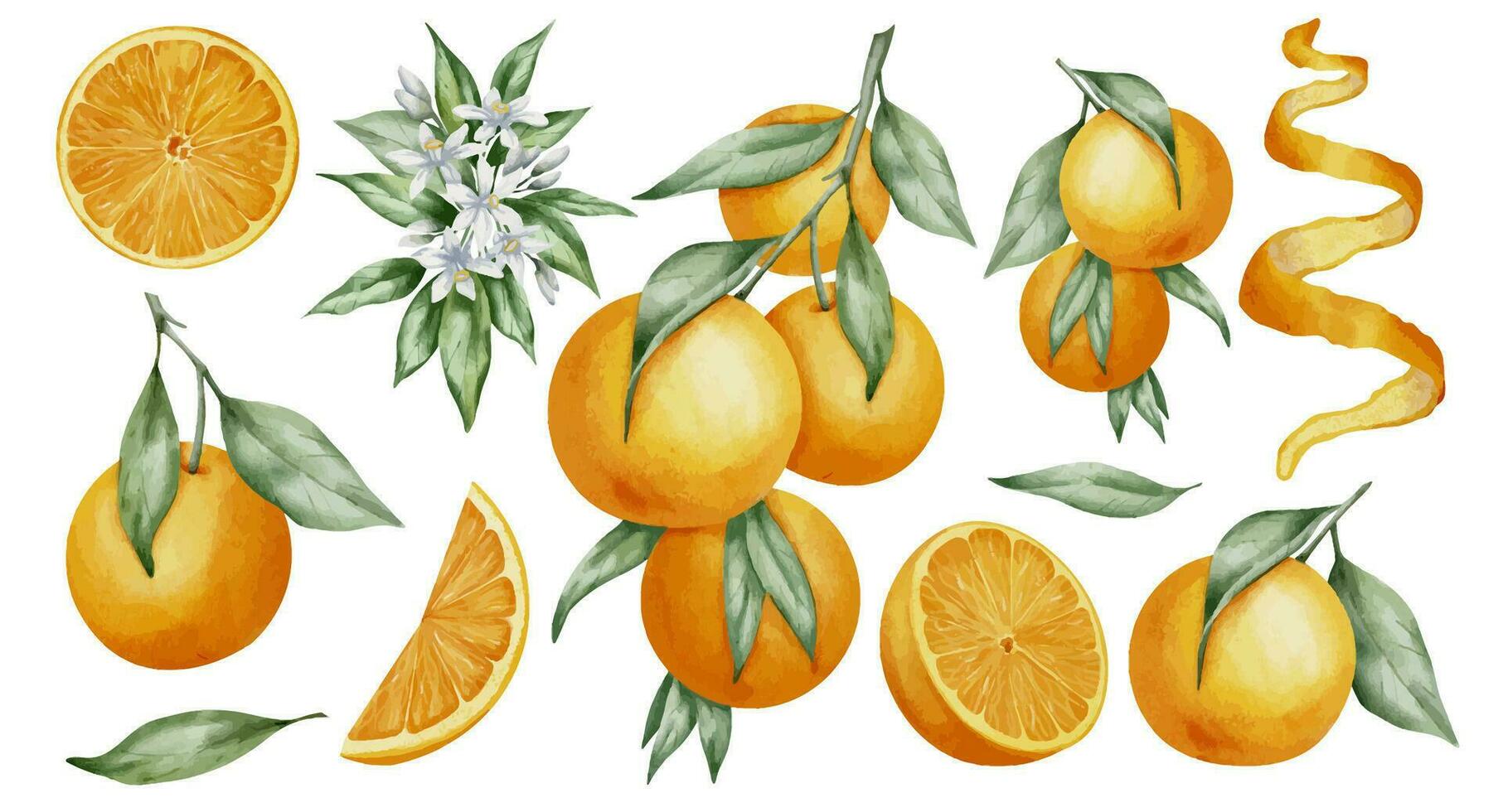This detailed color painting features a vibrant collection of oranges in various forms, arranged against a white background. In the top left corner, there's an orange slice facing us, displaying its segments. Below this, a whole orange is depicted with part of its stem and green leaves intact. To its right, another orange slice is positioned, showcasing its juicy interior. Nearby, a cluster of oranges with green leaves is situated on a branch adorned with white blossoms. To the lower right, an orange is cut in half, revealing its outer peel from a side angle. Above this, a pair of oranges hang from a stem. Additionally, there's an artistic swirl of orange peel depicted, creating a dynamic element in the composition. Toward the bottom right, another whole orange with a stem and two green leaves is present. The painting beautifully captures the natural diversity of oranges, emphasizing their rich colors and textures.